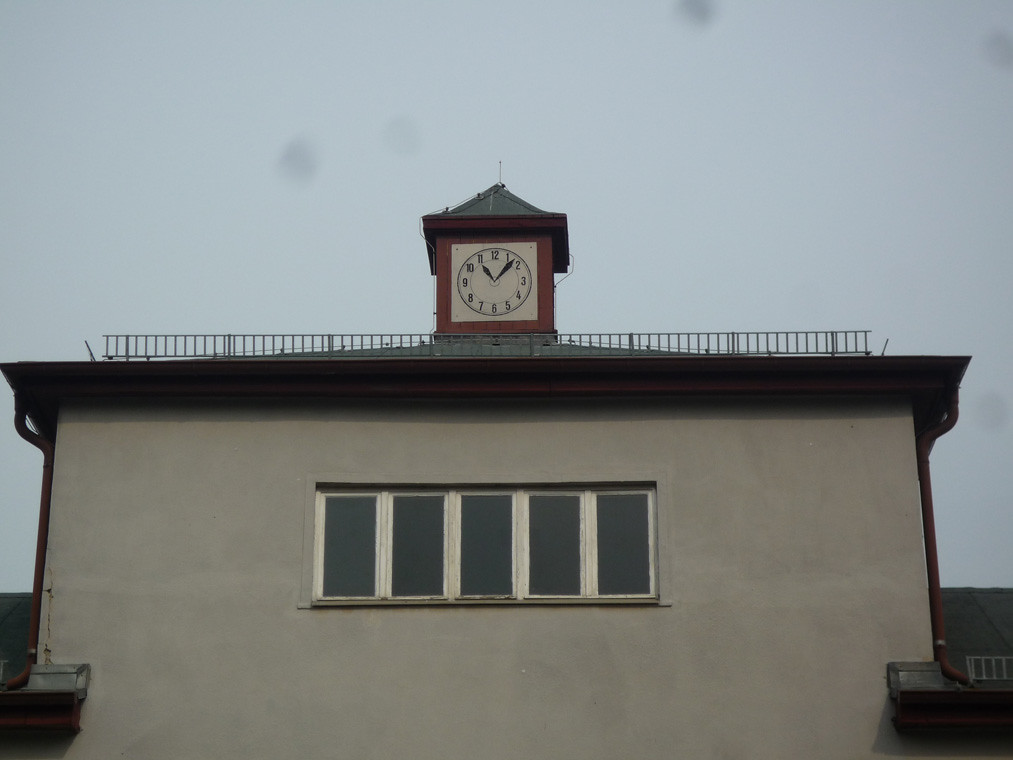This image captures a stucco-clad building set against an overcast sky so densely gray that individual clouds are indistinguishable, giving the impression of a uniformly cloudy day. The central focus of the shot is the middle section of the building, flanked on both sides by roofs featuring rust-colored gutters and eaves. Prominently positioned in the middle section are five windows arranged in a rectangular configuration. The building's architecture is further accentuated by an additional roof crowning the top section, framing a metal railing above. Perched atop the railing is an antique-looking clock with a rust-stained exterior and a tan face. The clock displays the time as 11:07 with striking black hands.